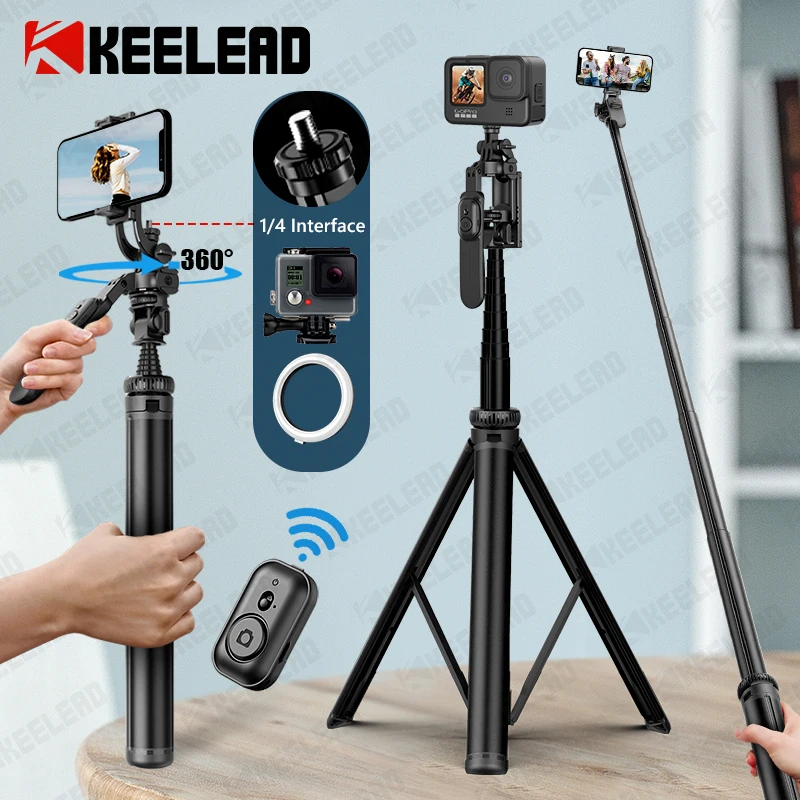The image prominently features three different types of camera stands against a light wood table and blue background. The top left corner of the photo displays the brand name "Keyland" in a large black font, accompanied by a logo with the letter "K" in a red square. The first camera stand on the left is a black pole with a short handle, held by two human hands, which has a cell phone clipped onto it. To the right, there is a traditional tripod with three legs, topped by a camera displaying an image of a person riding a motorcycle. The third stand on the right is a compact handheld camera holder. The image also includes details like a wireless remote control and writing indicating "360 degrees" and "quarter-inch interface" next to one of the tripods, suggesting advanced functionalities like a 360-degree swivel mount. The setup appears to be a product photo showcasing Keyland's range of photography tripods and accessories.